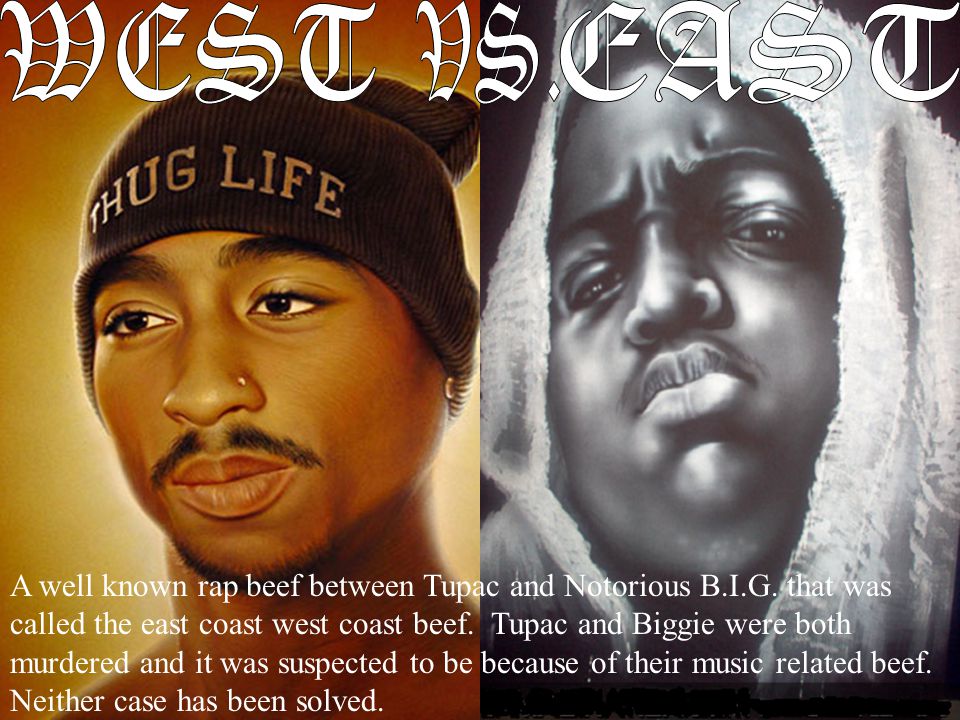This illustration features two prominent and deceased rappers, Tupac Shakur and Notorious B.I.G. (also known as Biggie Smalls), depicted in artistic renderings. On the left side, Tupac is shown in a three-quarter view, looking leftward, wearing a black beanie adorned with the words "Thug Life." The background behind Tupac consists of orange, yellow, and white hues. On the right side, Biggie is portrayed looking downward towards the viewer, with a white, fluffy hood draped over his head. His background is stark black. The image is split down the middle, symbolizing the notorious East Coast-West Coast rap feud. "West vs. East" is written in a challenging, ornate gothic font at the top of the illustration, while a detailed caption at the bottom in a white, italicized font reads: "A well-known rap beef between Tupac and Notorious B.I.G. that was called the East Coast-West Coast Beef. Tupac and Biggie were both murdered, and it was suspected to be because of their music-related beef. Neither case has been solved."